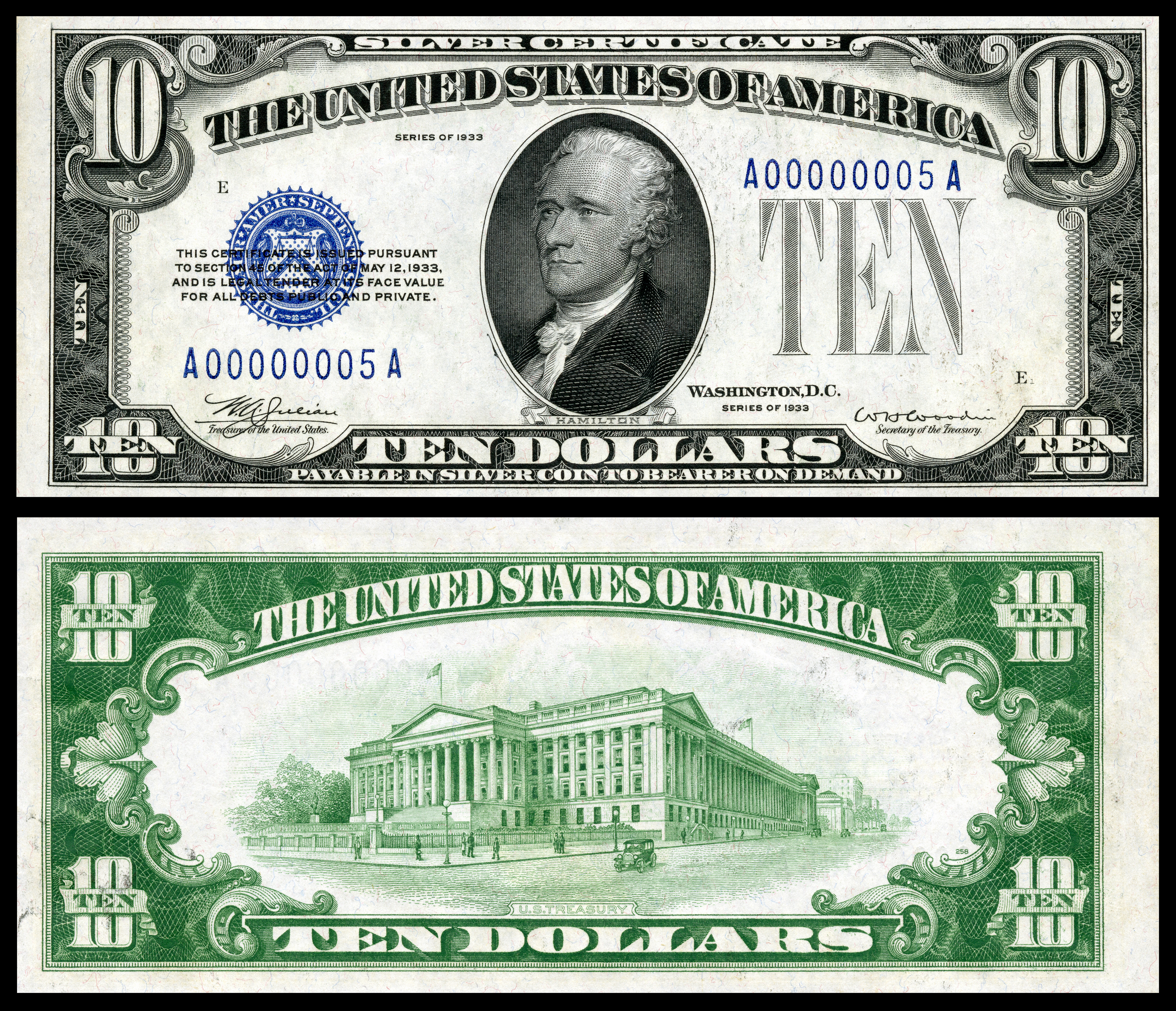This image portrays a historic $10 bill, specifically a Silver Certificate from the series of 1933. The photograph is divided into two sections: the top section features the front of the bill and the bottom section displays the back.

The front of the bill, primarily in black and white, prominently displays Alexander Hamilton at its center. The text "United States of America" crowns the top, while the denomination "10" is inscribed in each corner. Additional details include a blue seal of America on the left and a number "A00000005A" in the upper right corner. The phrase "$10 payable in silver coin to the bearer on demand" is clearly printed at the bottom.

The lower section of the image captures the back of the $10 bill, notable for its green and white color scheme. "The White House" is depicted in the center, surrounded by the text "The United States of America" and "10" in each corner. An old car can be seen on the road adjacent to the Capitol building, giving the viewer a glimpse into the historical context of the currency.